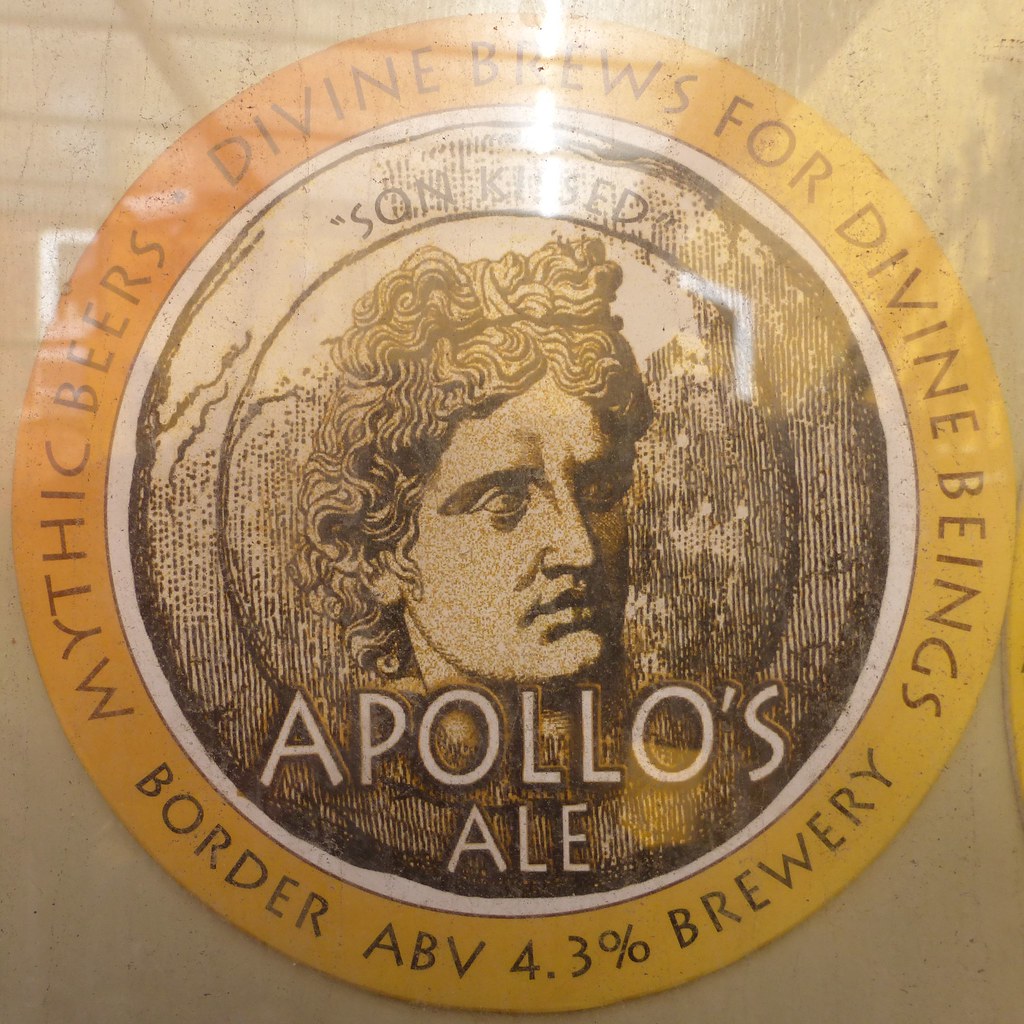The image showcases a central circular logo which appears prominently against a glossy, tan marble-esque background. Dominating the composition, the logo suggests either a beer cap or the side of a beer bottle. The focal point of the logo features what looks like an engraving or hand-drawn representation of Apollo, with a hatched texture suggesting detailed artistry. Above Apollo's head, partially obscured by a glare, the text "Sun-Kissed" is visible. Below, in larger white letters, it reads "Apollo's Ale." Encircling this central design is a border with the slogan "Mythic Beers, Divine Brews for Divine Beings," and at the bottom, it includes the name "Border Brewery" along with "ABV 4.3%." The color palette includes shades of tan, orange, black, gray, brown, and white, contributing to a rich, mythic aesthetic.